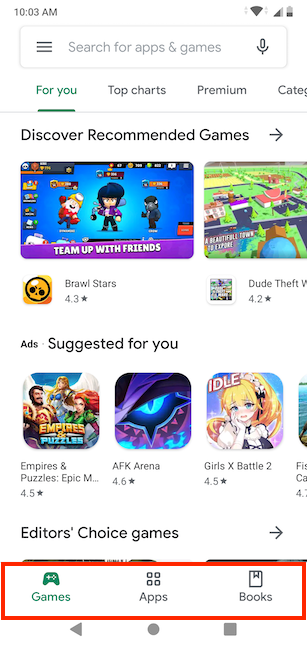In the image, we see a screenshot of a mobile app interface with the following elements:

1. **Background**: The background is white, providing a clean and uncluttered look.

2. **Header Section**: 
   - The time "10:03 AM" is displayed at the top.
   - To the right of the time, there is a small purple box featuring three horizontal stripes, commonly representing a menu icon for navigating apps and games.
   - A microphone icon is present, indicating voice search functionality.

3. **Navigation Tabs**: 
   - The tabs include "For You" (which is underlined, indicating the current selection), "Top Charts", "Premium", and "Categories".

4. **Content Section**:
   - The section begins with "Discover Recommended Games" and a left arrow icon, suggesting navigable content.
   - Below this header are featured game listings, starting with:
     - **Brawl Stars**: Accompanied by an icon of a skeleton head outlined in black with yellow and red detailing. A brief description reads "Team up with friends".
     - **Dude Theft V**: Rated 4.2 stars.
   - An ad labeled "Suggested for You" includes:
     - **Empires & Puzzles**: Rated 4.5 stars.
     - **AFK Arena**: Rated 4.6 stars.
     - **Girls X Battle 2**: Rated 4.5 stars.
   - Partially visible content indicates more recommendations and suggests that the list continues.

5. **Editors’ Choice**:
   - The section includes "Editors’ Choice Games" with a right arrow icon, indicating more options available to view. Some text is cut off, hinting at additional content.

6. **Navigation Bar**:
   - At the bottom, there is a red square divided into "Games", "Apps", and "Books".
   - Common navigational icons of a triangle, circle, and square are also displayed, representing typical mobile navigation buttons.

This detailed description encapsulates the various elements presented in the screenshot, providing a comprehensive overview of the interface.